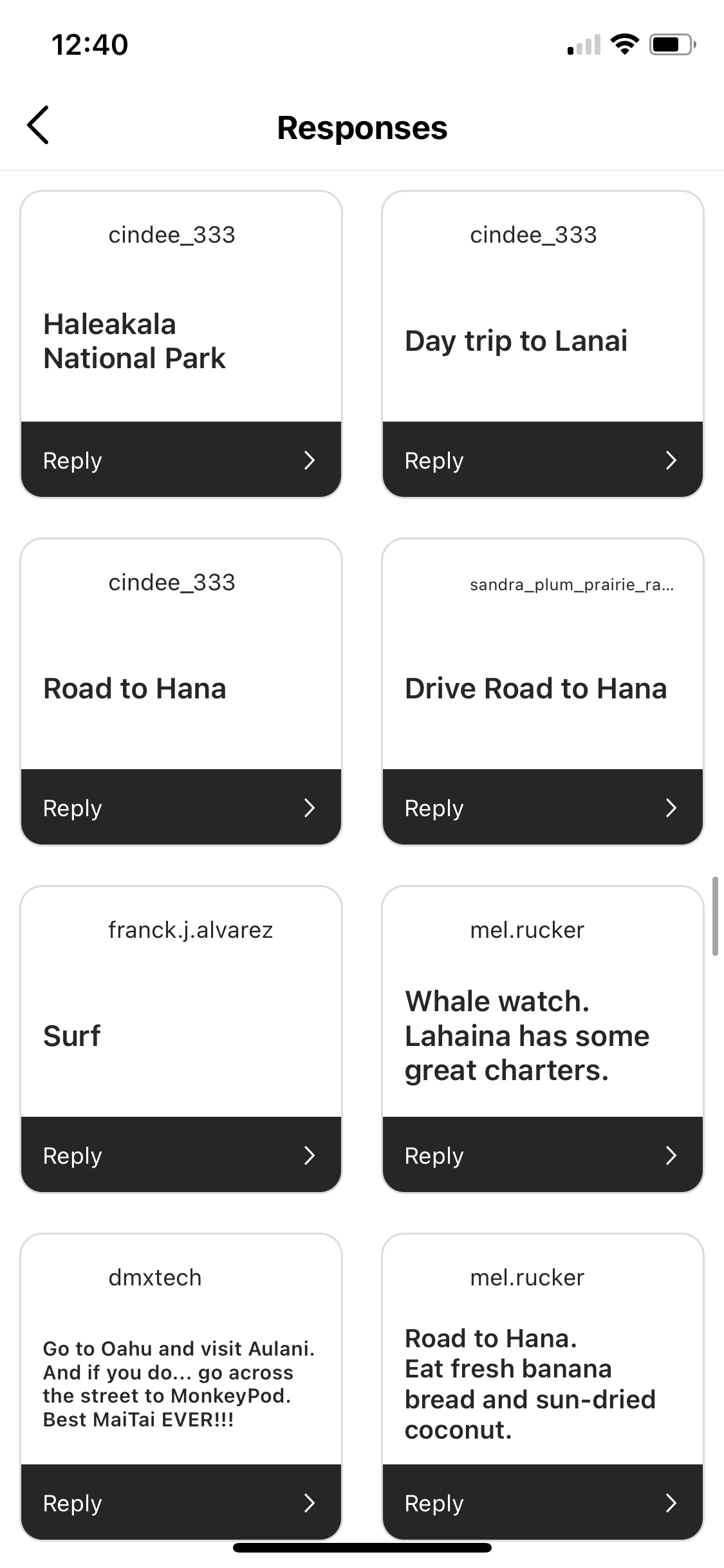**Detailed Caption:**

A close-up screen capture of a cell phone displaying an app interface. The top ribbon of the phone screen features standard icons: the time on the left and indicators for battery life and signal strength on the right. Below this ribbon, the app interface consists of a grid layout with two columns of four rows of white square message blocks, each outlined with rounded corners and containing black text. 

The upper left block reads "Halika National Park," adjacent to it on the right, the block says "Day Trip to Lahina." The second row starts with "Road to Hana" on the left, and "Drive Road to Hana" on the right. The third row contains "Surf" on the left and "Whale Watch" on the right, accompanied by a note: "Lahana has some great charters." 

In the final row, the left block mentions "Go to Oahu and visit AULANI. And if you do, go across the street to Monkey Pod. Best Mai Tai ever." The block to the right initially says "Road to Haha" but corrects to "Road to Hana, H-A-N-A," adding a suggestion to "Eat fish, banana bread, and sun-dried coconut."

At the very top of the screen, above the grid, there's a heading titled "Responses" and each message block includes a reply button at the bottom. The text is straightforward, with no additional color accents, maintaining a clean, monochromatic design.